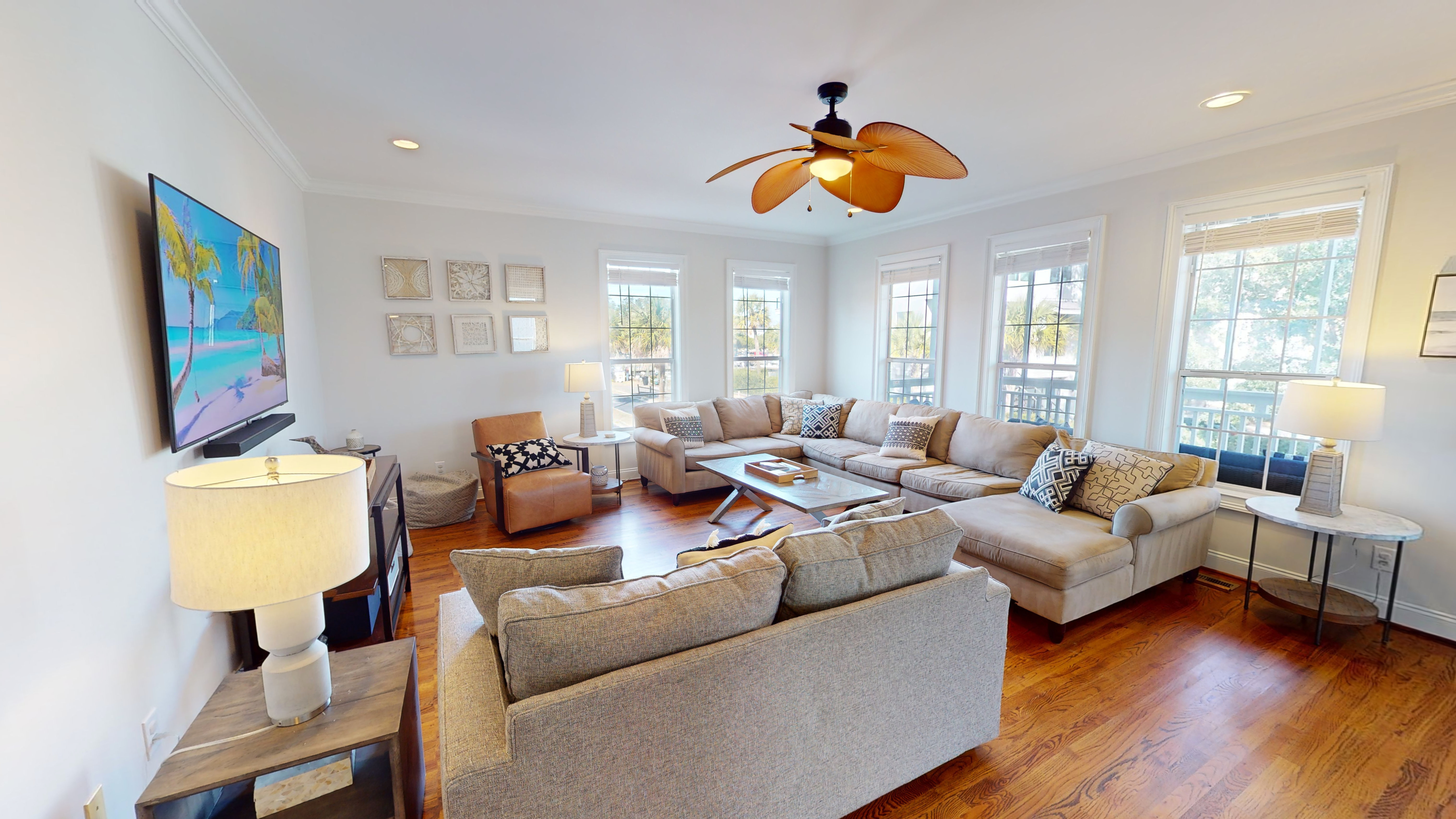This photo captures a well-lit living room with a warm and inviting ambiance. The hardwood floor and white walls create a clean, modern backdrop, while the ceiling fan with five brown, leaf-like blades, which is adorned with gold chains, provides a touch of elegance. The fan is complemented by additional ceiling lights embedded within the white ceiling. A large sectional and a gray loveseat dominate the seating area, both dressed with an array of mostly white, black, and tan pillows, contributing to the room's cozy feel.

At the left-hand side of the room, a sizable flat-screen TV, showing a beach scene, is mounted on the wall with a sound bar beneath it. In the foreground, a brown chair with a white and black pillow adds another seating option. Three tables spread throughout the room hold various lamps: one in the left-hand corner with a white cord and off-white lampshade, a white table in the middle back featuring a similar lampshade with black legs and base, and another white table on the far right with a white or brown lamp and a shelf underneath.

Natural light streams through five large windows at the back of the room, highlighting black fencing and lush green trees outside. Additionally, the room features six decorative wall pictures in a horizontal row near the windows. Each of these elements, from furniture placement to the strategic lighting, contributes to a harmonious and thoughtfully arranged living space.